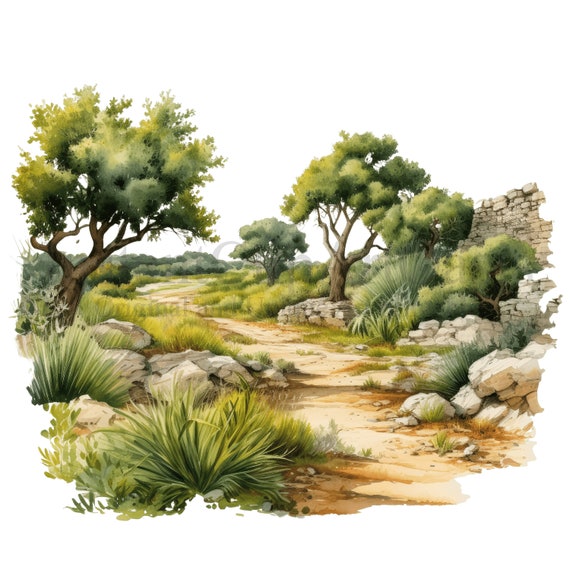This illustrated image depicts a winding dirt path with a slight incline, meandering through a picturesque landscape framed by a rich variety of vegetation and geological features. The path, rendered in tan and brown hues, is flanked on both sides by clusters of tall grasses, lush green trees with full canopies, and bushes. Scattered among the flora are numerous large boulders and rocks, enhancing the rugged beauty of the scene. 

On the far right side of the image, the remnants of what appear to be human-made stone formations or walls are visible, hinting at past structures. The sky above is an expanse of white, contrasting with the detailed, natural elements below. Adding to the unique artistic style, the edges of the painting are not confined to a traditional square; instead, the borders follow the organic contours of the plants and landscape, creating a jagged frame that emphasizes the natural setting.